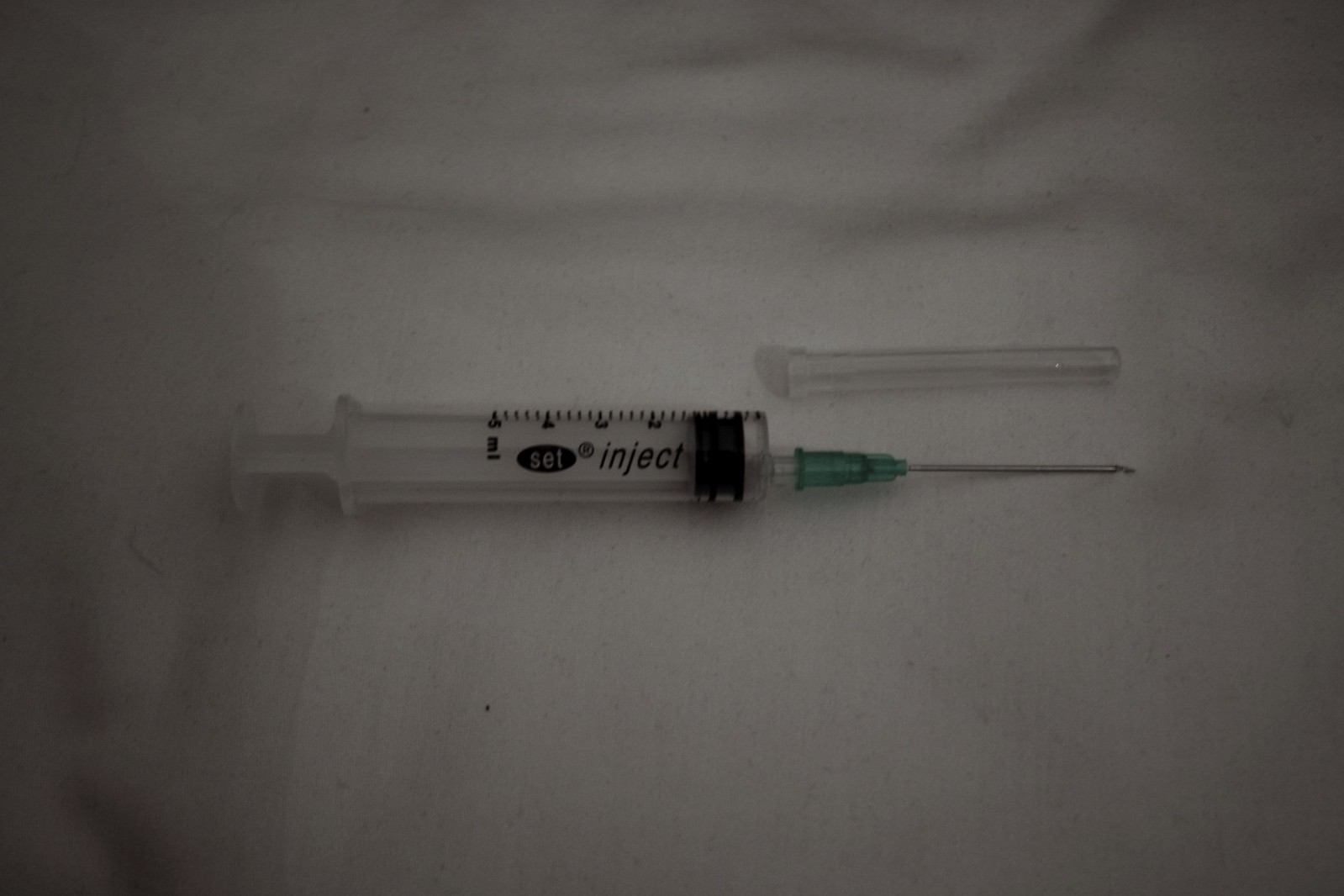This is a detailed photograph of a hypodermic needle, positioned horizontally on a slightly wrinkled white cloth. The needle tip is pointing to the right, with the base of the syringe to the left. The plastic needle cover has been removed and is placed on top of the needle. The needle is connected to the syringe with a green plastic part, transitioning into a black and clear body. The syringe is marked with a scale ranging from 1 to 5 milliliters, and it features the brand "Set" with a trademark symbol (®) as well as the word "Inject" in italic letters. The surface beneath the syringe is a bit blurry, but the prominent details of the syringe are clearly visible against the white background.